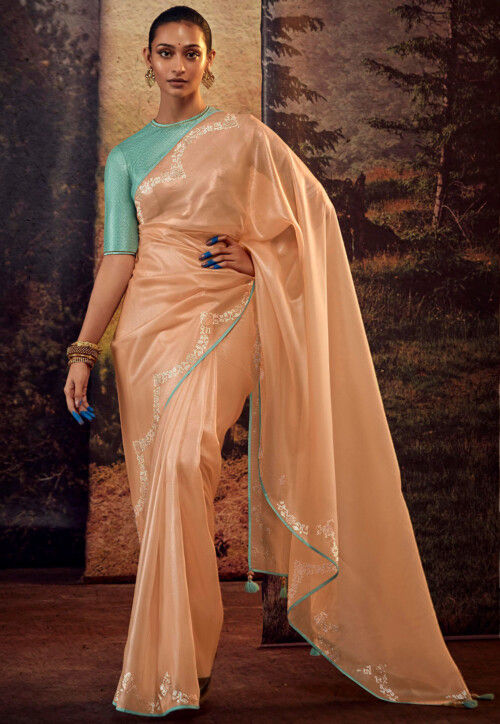This photograph captures a stunning young woman of Indian descent, elegantly modeling an exquisite sari. The ensemble features a luxurious, salmon-colored sari made from shimmering silk or satin, which drapes dramatically over her left shoulder and cascades to the floor. The sari is accentuated by turquoise piping and delicate tassels, with intricate golden embroidery or beadwork along its edges. Beneath the sari, she wears a vibrant teal blue top with elbow-length sleeves. Her accessories add a touch of glamour, including bulky gold bracelets, matching earrings, and a bindi on her forehead. Her long fingernails, painted in a striking blue, complement the attire. Her hair is sleekly pulled back into a bun, contributing to her clean and sophisticated appearance. She stands against a backdrop of dark, tapestry-like fabric depicting a forest scene, adding an extra layer of richness to the composition. With a neutral expression and one hand poised on her hip, she embodies grace and timeless elegance, suggesting she is prepared for a formal event or celebration.